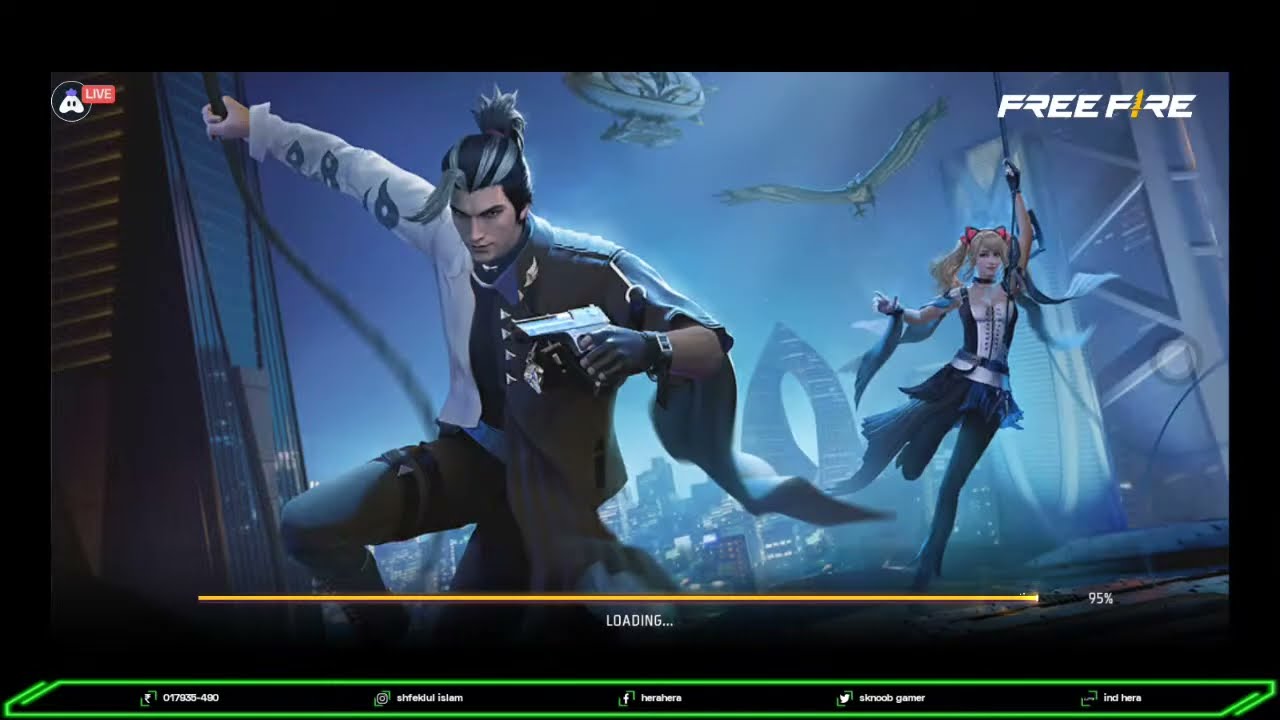The image appears to be a loading screen from the video game "Free Fire," indicating 95% loading progress with a yellow bar and the word "Loading" beneath it. On the top right corner, the game's title "Free Fire" is prominently displayed. The scene features an animated man and woman, both engaging dynamically with ropes. The man, positioned on the left, has dark hair tied in a ponytail with white streaks, and he is seen holding a gun while kneeling, suggesting he has just flown through the air. He wears a cape-like shirt and pants, adding to his adventurous appearance. To his right, the woman is dressed in a silver corset with buttons, a short skirt, black tights, and has her hair styled in pigtails adorned with ribbons. She also holds a rope, appearing to have just landed with one foot on the ground. Behind her, a bird with long wings is visible, and the backdrop includes a cityscape with skyscrapers and girders. On the top left corner of the screen, it indicates "Live" on a red background, likely referring to a live stream, along with various social media icons and handles related to the streamer at the bottom of the screen within a neon green rectangle.